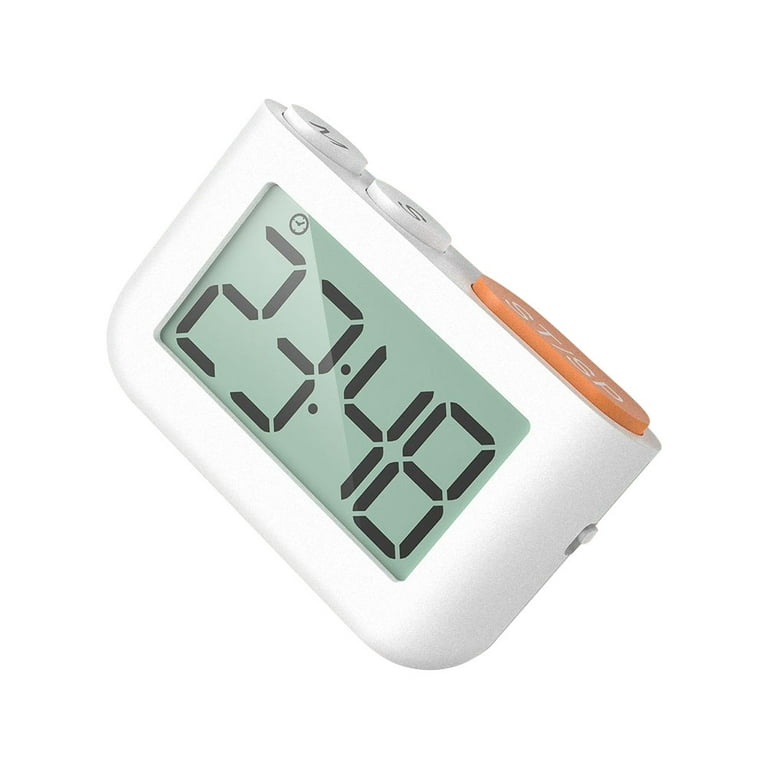The image depicts a modern digital timer or alarm clock, angled diagonally at approximately 45 degrees against a pure white background. The device is white and rectangular, with a predominantly plastic case and an oblong shape. The large digital display, set against a light grayish or bluish LCD background, clearly shows the time as "23:48," indicating a 24-hour format. Below the display, there are three buttons on the top: a "M" button for minutes, an "S" button for seconds, and a larger orange or red "ST/SP" button for start/stop. Additionally, a small, unmarked switch is located to the right, possibly for changing the time format or toggling an on/off function. In the upper left corner of the display, a small LCD icon of an alarm clock is visible, though its function is unclear.